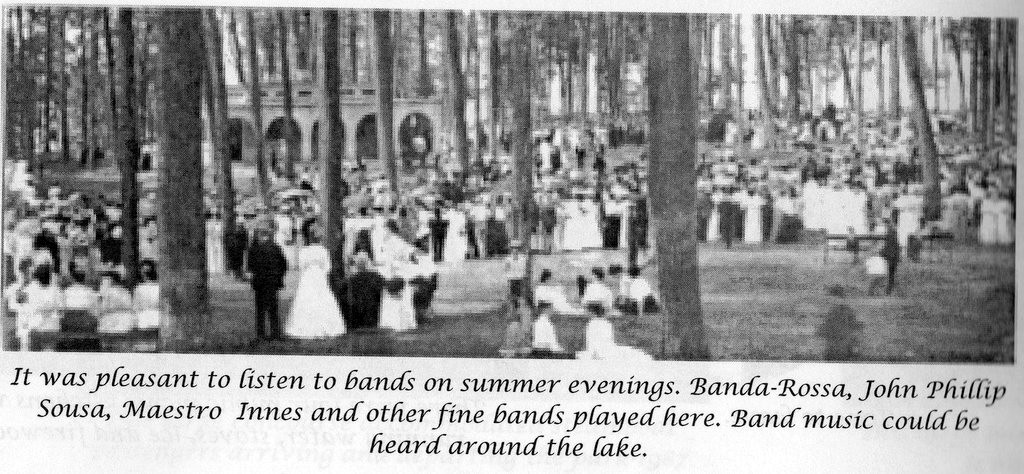This grainy black and white photograph captures an outdoor setting with a large field surrounded by many tall trees, their trunks prominently visible. Numerous people, including men in black suits, women in long dresses, and some children in white outfits, are gathered on the grass. In the background stands a building with five arch entrances. Below the photo, text in black letters reads: "It was pleasant to listen to bands on summer evenings. Banderosa, John Philip Sousa, Mastro Ennis and other fine bands played here. Band music could be heard around the lake."